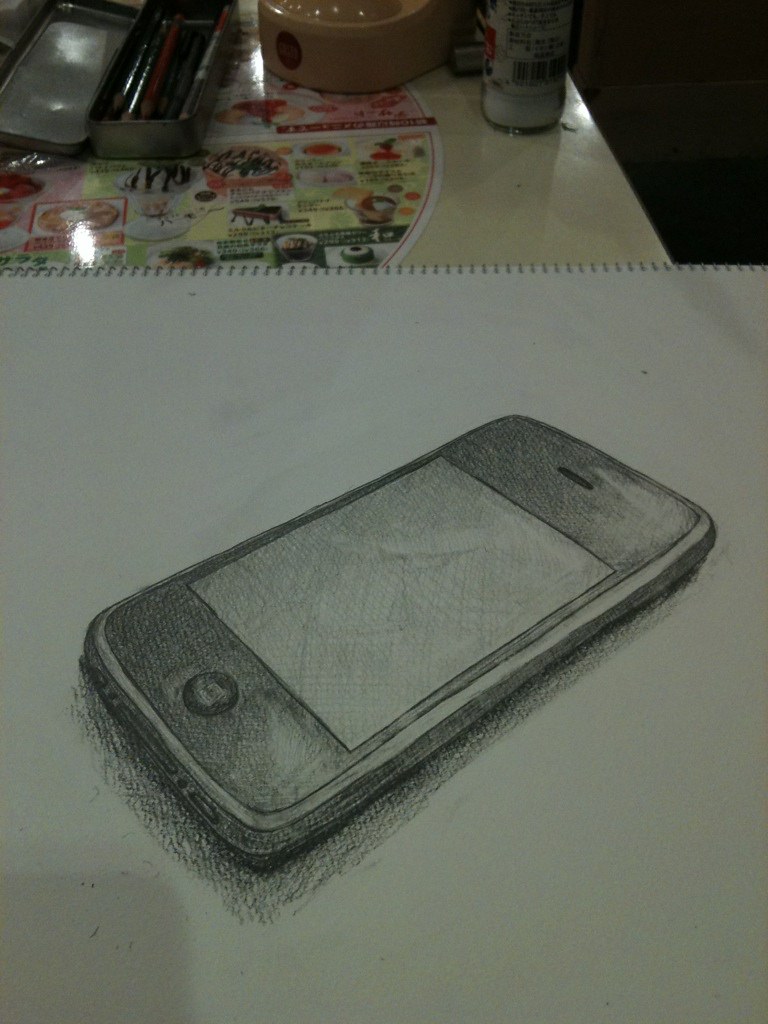A meticulously rendered pencil drawing of a cell phone takes center stage in this image, resting atop a plain paper spiral-bound notebook on what appears to be a restaurant or coffee shop countertop. To the left, a vibrant placemat adorned with dessert menu items adds a splash of color, hinting at a sweet indulgence locale. In the blurred background, a can of indeterminate purpose, a utensil-filled box, and a mysterious orangey-brown object punctuate the scene, providing a cozy yet cluttered backdrop.